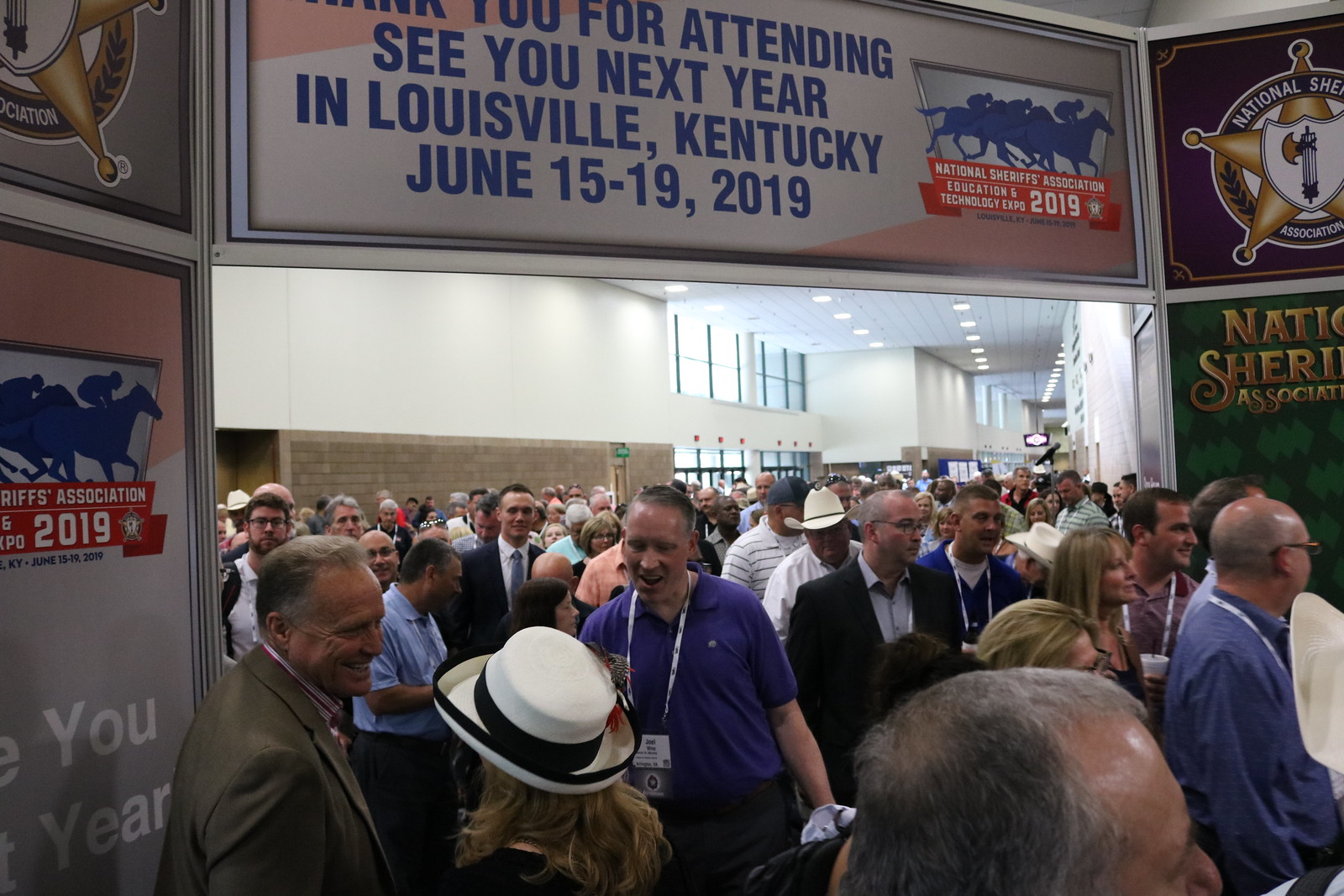The photograph depicts a busy scene at the National Sheriff's Association Conference, held indoors within a convention hall or venue linked to Churchill Downs, renowned for the Kentucky Derby. A large crowd, predominantly Caucasian, is moving through a wide doorway into the main area, with many attendees wearing hats, suits, and passes around their necks. Overhead, a prominent sign reads, "Thank you for attending. See you next year in Louisville, Kentucky, June 15-19, 2019," accompanied by a banner featuring horse racing imagery and the National Sheriff's Association logo. The walls are adorned with various advertisements and banners, including a green billboard and a red background sign that reads "National Sheriff's Association Education Technology Expo 2019," as well as several depictions of blue jockeys. The scene is vibrant and colorful, with attendees wearing a variety of clothing in black, blue, and white, while moving in one direction through the crowded hallway. Notable details include a woman with a white hat trimmed with a black ribbon and the visible sheriff's badge logos that underscore the event's official theme.